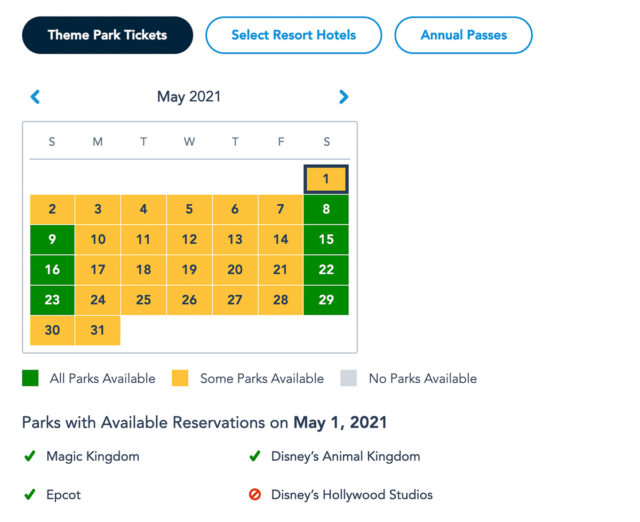The webpage is designed for purchasing theme park tickets and features a navigation bar at the top with three distinct buttons. The first button, labeled "Theme Park Tickets," has a dark blue background, while the next two buttons, "Select Resort Hotels" and "Annual Passes," have white backgrounds with blue text.

Below the navigation bar is a calendar for May 2021, displayed in a standard weekly format: SMTWTFS. The first day of May is outlined in blue, while most other dates are yellow. Weekends are highlighted in green, except for May 30th, which remains yellow.

Underneath the calendar, a legend explains the color coding: a blue square signifies "All Parks Available," a yellow square indicates "Some Parks Available," and a grey square means "No Parks Available."

Further down, there's a section titled "Parks with Available Reservations on May 1st, 2021." Here, Magic Kingdom, Epcot, and Disney's Animal Kingdom each have a green checkmark next to their names, indicating availability, while Disney's Hollywood Studios has an icon of a circle with a line through it, suggesting no availability.